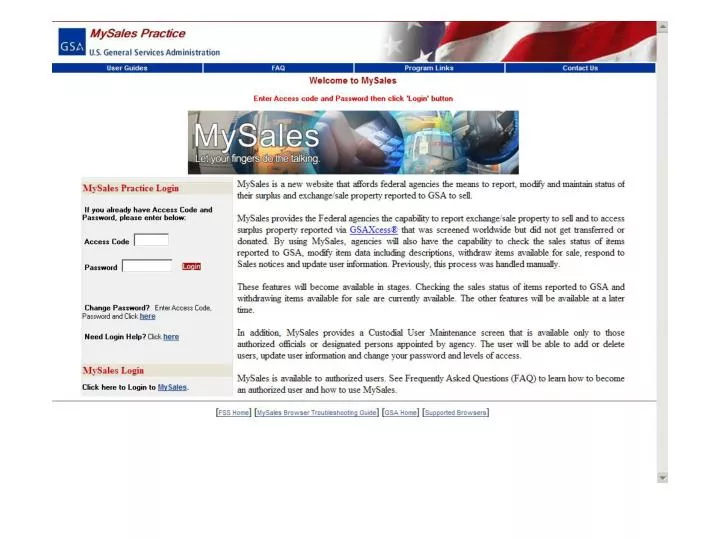The image depicts a practice screen for the U.S. General Services Administration's "MySales" application. The term "MySales" appears as a single word with both the 'M' and 'S' capitalized and highlighted in red. Beneath it, in smaller blue text, reads "U.S. General Services Administration."

On the left side of the image, there is a blue box featuring the GSA logo in white. Adjacent to it, on the right, there's a watermark displaying a picture of the United States flag. Below the "U.S. General Services Administration" text, four clickable buttons are arranged for user guidance: "User Guide," "FAQ," "Program Length," and "Contact Us."

Centrally located on the screen, a red heading welcomes users to "MySales" and instructs them to "Enter access code and password then click login." Complementing this, a white box beneath displays the slogan "MySales: Let your fingers do the talking," accompanied by 3D-rendered images that suggest a user typing.

Towards the lower left of the image, a gray box titled "My Login Information" prompts existing users to enter their access code in a designated field. There is also a password field and a red "Login" button. Below this, options for changing the password and an additional login button appear in blue text.

The bottom section of the screen provides a detailed explanation of the "MySales" website, emphasizing its role in allowing federal agencies to report, modify, and maintain their status or surplus information. Additionally, links for "FSS Home," "Troubleshooting Guide," "GSA Home," and "Supported Browsers" are present at the very bottom of the screen for further navigation.